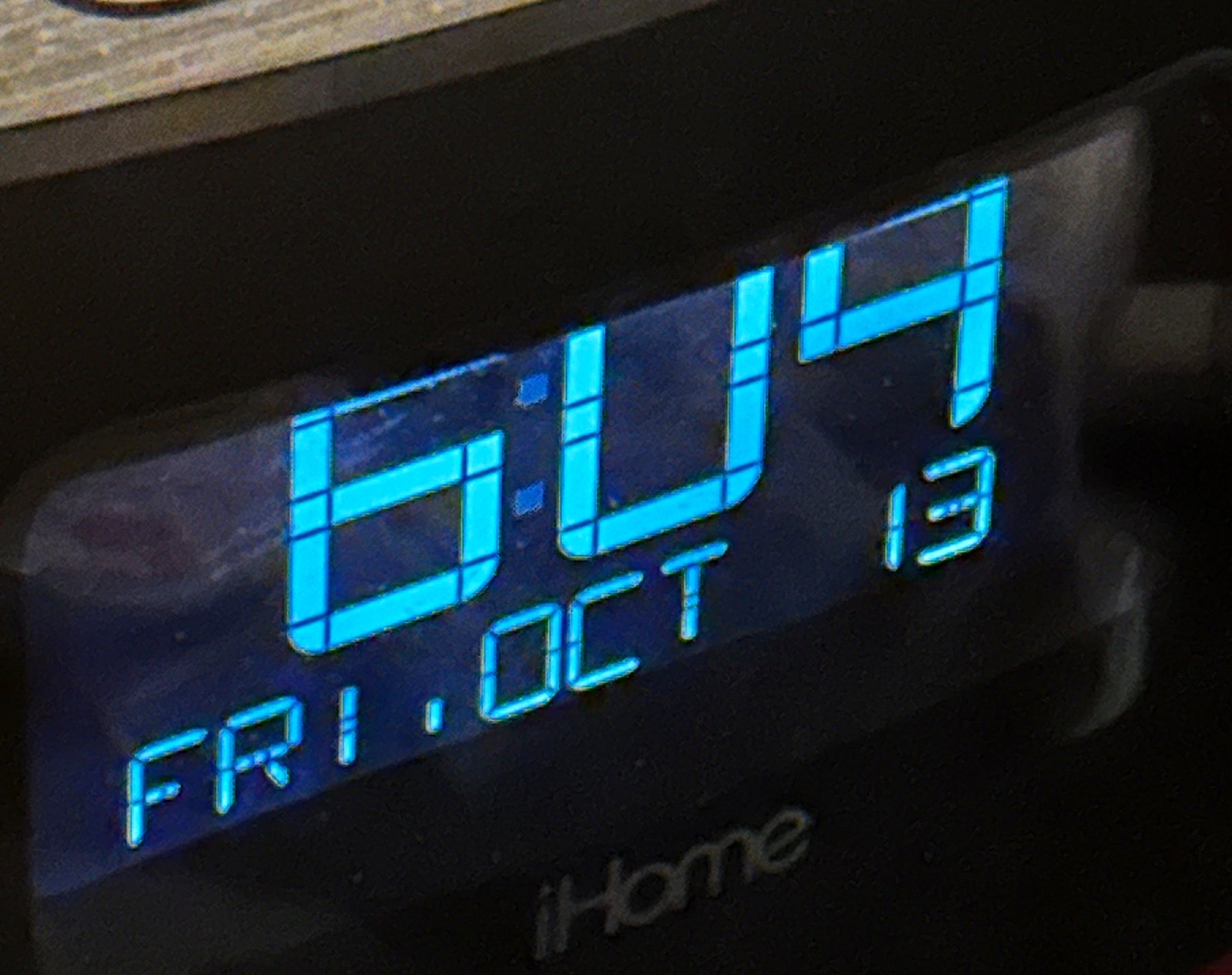This image is a close-up, slightly angled photograph of a black iHome digital alarm clock. The iHome brand logo is prominently displayed at the bottom in white letters, with the distinct styling of a lowercase "i" followed by an uppercase "H" and then lowercase "ome." The clock's large screen emits a blue glow, and it's currently displaying the time as 6:09. Just below the time, in smaller light-blue alphanumeric characters, the clock indicates "FRI, OCT 13." The photograph is darkly lit and appears slightly out of focus, adding a blur effect to the overall image. The upper left corner reveals a small triangle of striped carpet, suggesting the clock is positioned close to the ground. Light reflecting off the front of the clock accentuates its glossy finish.